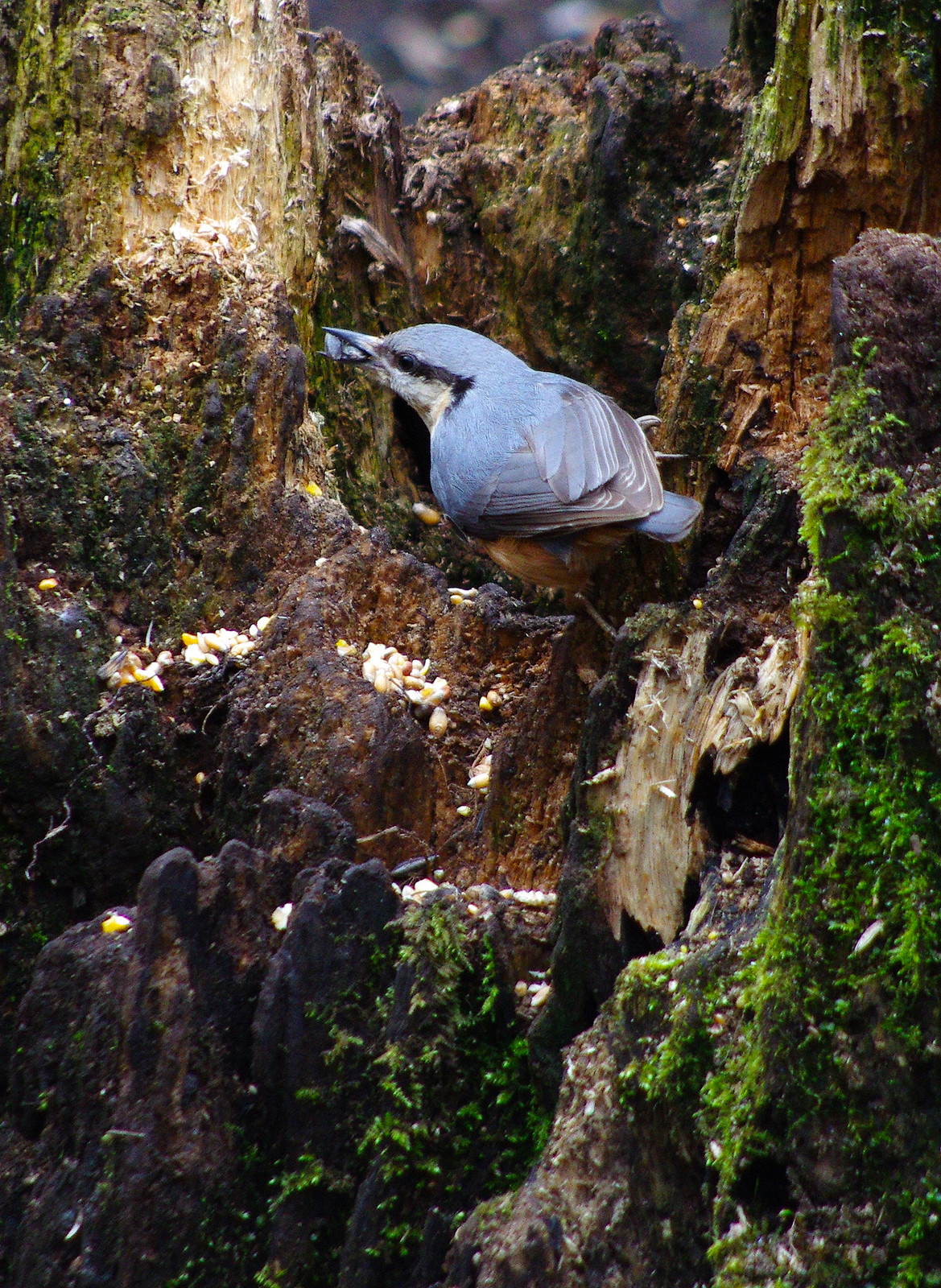This vivid photograph captures a small bird perched within the rotting remains of a tree trunk. The bird, a delicate blend of light blue and gray feathers with distinct black markings, is positioned at the center of the image. Its underside is white, and a striking black stripe runs from its beak, past its eyes, and towards its body. In its black beak, the bird clutches an oval-shaped bug, possibly preparing to enjoy its meal. Surrounding the bird at the base of the tree trunk is a pile of acorns and multiple round, white insects and bugs, suggesting a bustling micro-ecosystem. The wood of the tree is visibly deteriorated, with sections scraped off and patches of green moss adding to the natural beauty. There's no human presence in the photo, allowing the focus to remain entirely on the bird and its surroundings. The background beyond the tree trunk is softly blurred, providing a serene and picturesque setting.